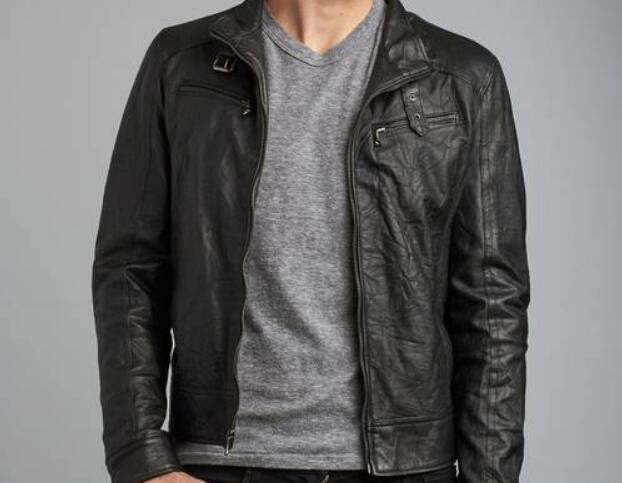In this close-up image from the waist to the neck, a Caucasian man stands against a light gray wall, displaying a simple, yet detailed ensemble. His attire includes black jeans and a slightly speckled charcoal gray crew neck t-shirt. Over this, he dons a worn, black leather jacket that remains unzipped, revealing the subtle crinkles and stitch work of the material. The jacket features zippered pockets on each breast and a buckle strap around the collar designed to fasten for added warmth on cold or windy days. Only a sliver of his neck and a bit of one hand is visible, showcasing his minimal, straightforward style.